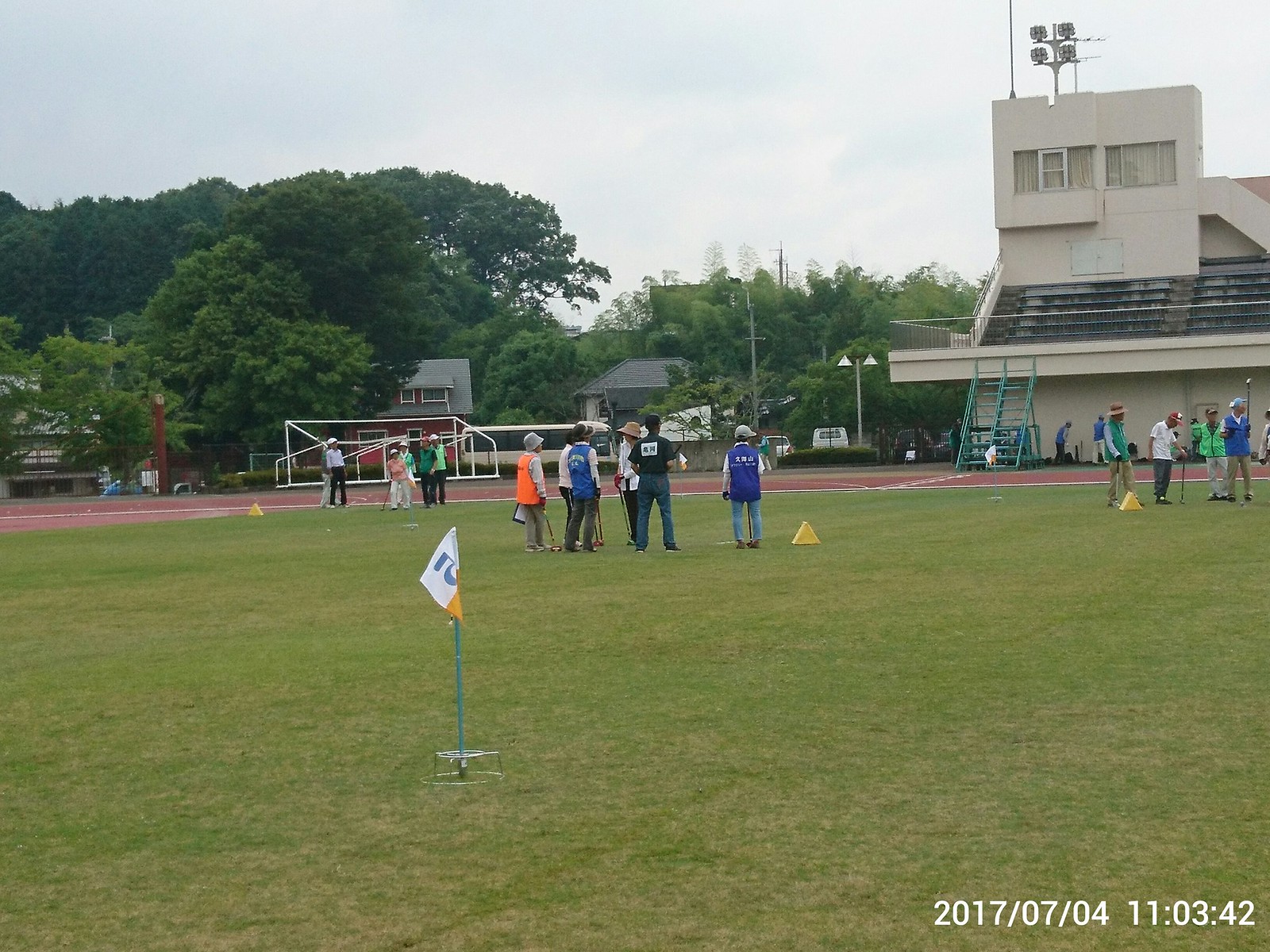The image showcases a large outdoor field, surrounded by a red and white track with white stripes, likely part of a school stadium. In the upper right-hand corner, there is a white stone building with attached floodlights and bleachers beneath a sky filled with a blend of white and gray clouds. On the left-hand side stand tall green trees, with shorter trees in the middle. Scattered across the grassy field are groups of people, many holding what appear to be sticks, possibly golf clubs. They are wearing various vests in blue, orange, and green, accompanied by jeans; some are also wearing hats. The right side of the field shows additional groups of people, with the background depicting homes, cars, a bus, and further large green trees. Closer to the camera, there are yellow triangular markers and a flag on a metal frame. The bottom right corner of the image displays the date and time: 2017/07/04 at 11:03:42.